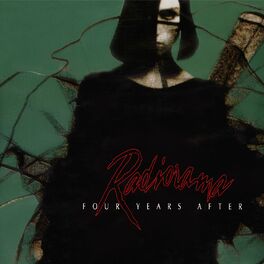The image is a possible album cover featuring a woman with very dark, shoulder-length hair that almost completely covers one side of her face, revealing only her left eye and pouted lips. Her expression is very serious, and her face is notably pale with dark eyes and pronounced shadowing along her cheek. She is wearing a black dress or top, and there are various dark shapes and ribbons intertwined around her and possibly in her hair. The background is a dark green with a brown, ribbon-like object cutting through the scene and what appears to be the tip of a bat extending out from behind her left shoulder. There is text on the image, reading "four years after" in white, preceded by an indistinct word in red, possibly related to the album's title.